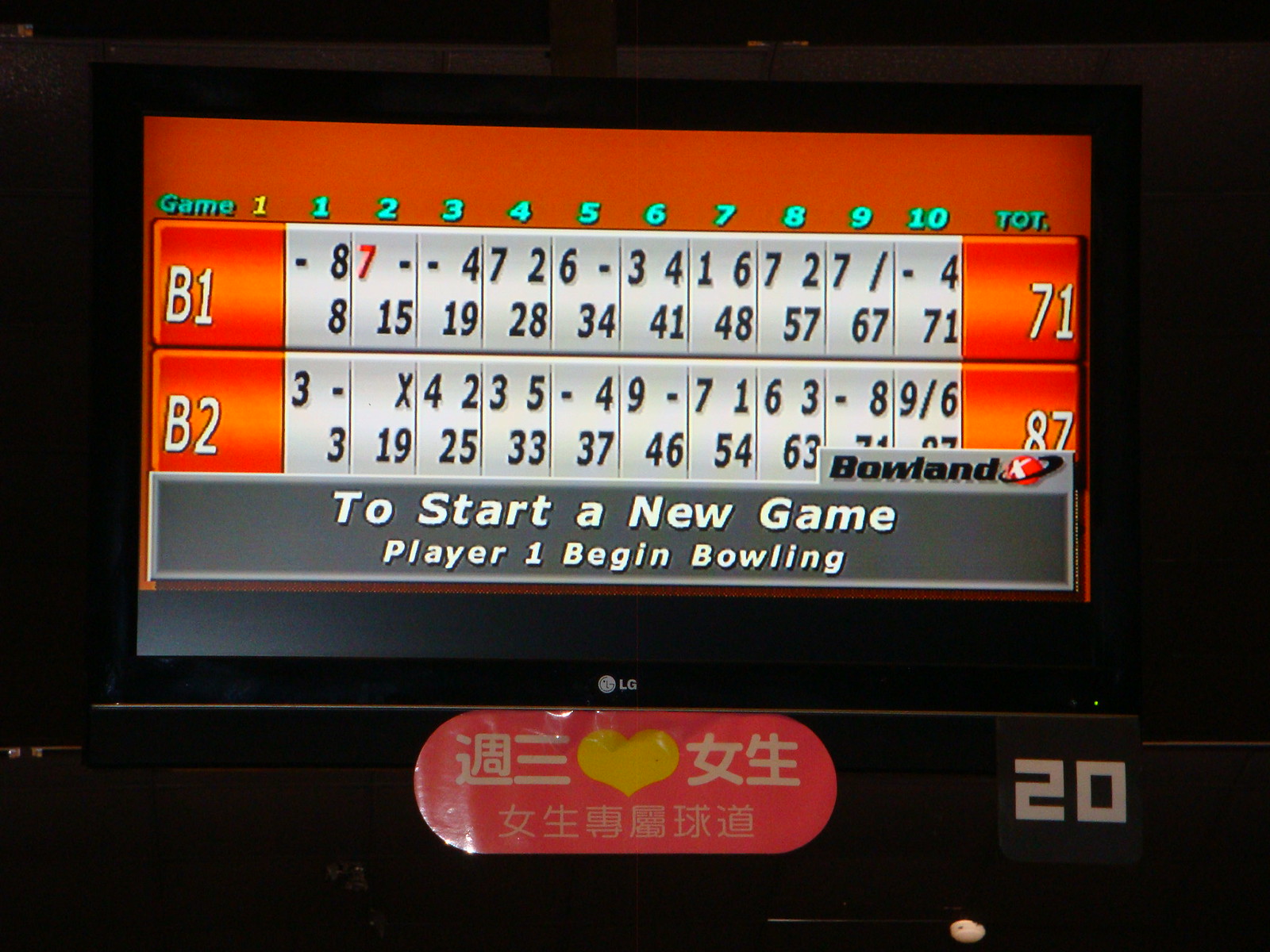The image shows a digital bowling scorecard displayed on an LG TV screen. The background of the scorecard is predominantly orange-red, and it features various columns labeled "Game" with each game numbered from 1 to 10 in green or teal ink, followed by an additional column marked "TK2." Below these columns, there are rows for two players, labeled "B1" and "B2," each containing their respective scores. In the first game, Player B1 has a total score of 71, while Player B2 has 87. The TV screen reflects some light at the bottom, highlighting the LG logo in the lower-left corner. The overall scene appears to be dimly lit, enhancing the prominence of the TV screen. At the bottom of the scoreboard, there's a gray box with instructions: "To start a new game, Player One begins bowling." Additionally, there is a red sign with Japanese lettering underneath the scoreboard.